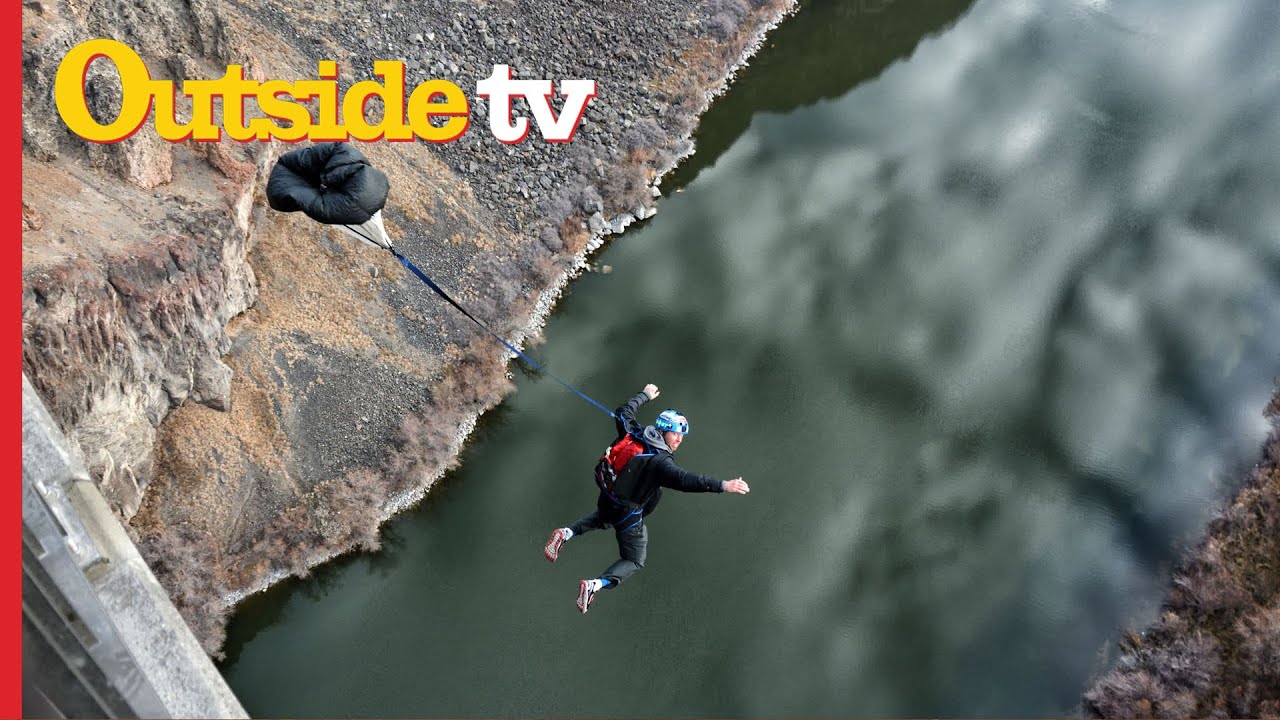In this image capture for the TV channel "Outside TV," the label is prominently displayed at the upper left corner, with "Outside" in yellow and "TV" in white bordered by red. A person is featured mid-air having just deployed a parachute, showcasing a thrilling skydiving moment. The individual, wearing a blue helmet, green pants, white and red sneakers, and a red and black backpack, looks back towards the camera. The parachute is black with a blue cord. The backdrop features cliffs and a bridge frame made of concrete. Below, the terrain appears photoshopped, with green and gray hues resembling water and brown rocky patches, adding to the dramatic nature of the scene.